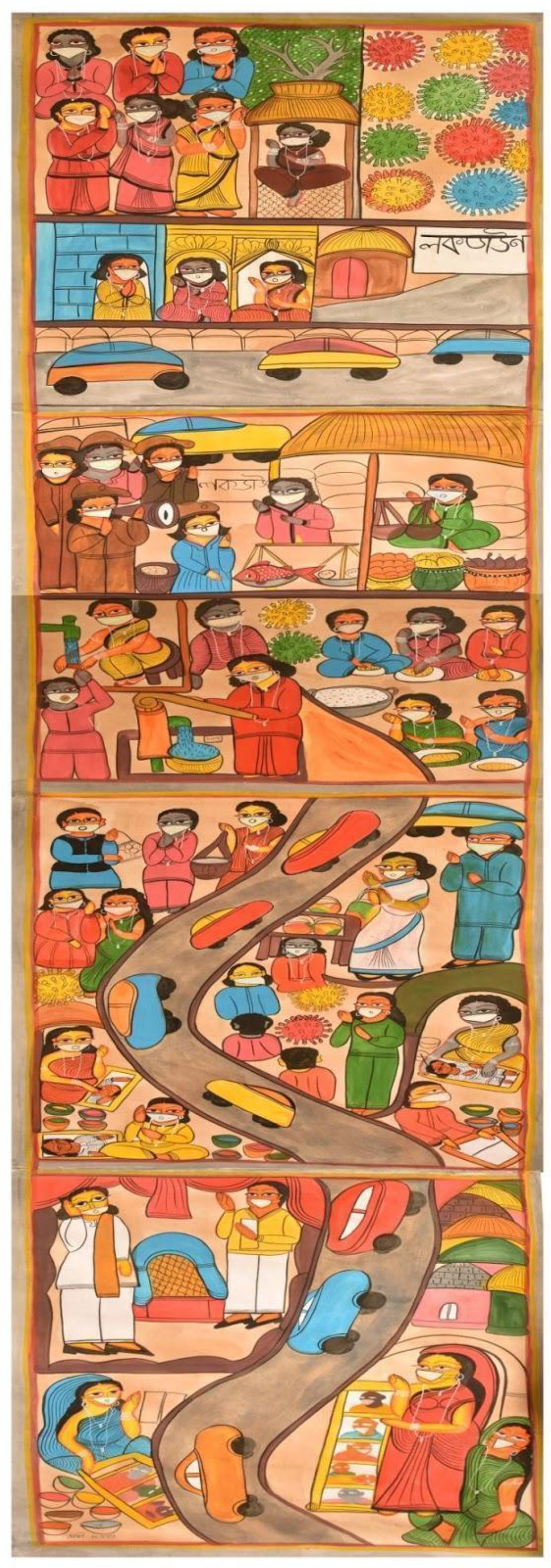The image is a detailed, hand-drawn artwork reminiscent of illustrations for a children's book, characterized by its vivid, childlike quality and vibrant colors. It is vertically rectangular and divided into several horizontal panels, layered to suggest a continuous scene. The drawing features an orange border and is set against a white background, giving the appearance of a wall hanging or tapestry.

At the top of the image, there are six people, presumably Asian, depicted in bright clothing and wearing white face masks, with the distinctive shape of the COVID-19 virus illustrated in greens, yellows, blues, and reds to the right. Moving downward, the middle panels show more masked individuals at a marketplace, surrounded by simple, colorful illustrations of fruit, vegetables, and fish, indicating a lively market scene.

In the panels below, people are gathered, possibly engaging in food preparation or a social gathering, again all wearing masks. The bottom half of the drawing depicts a winding roadway forming an S-shape, populated by basic yet brightly-colored cars in red, blue, yellow, and orange hues. The road is bordered by more onlookers in masks. The entire scene appears lovingly crafted with a crayon-like texture, giving it an endearing, innocent charm as if created by a talented child.